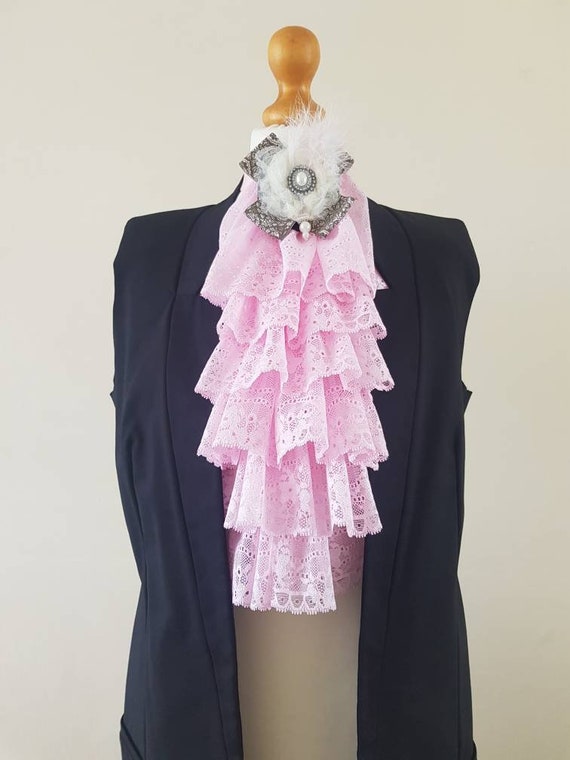This image features a partially finished black dress displayed on a wooden mannequin. The dress, resembling a suit vest and extending to about hip length, is paired with a prominent, frilly pink lace cravat that resembles a scarf with multiple ruffled sections. The cravat is adorned with a silver pin and needle, encircled by delicate white feathers and a pearl-like ornament in the center. The mannequin’s wooden top is tan-colored. The background is a nondescript, blank cream or beige wall, enhancing the contrast between the black dress and the intricate pink lace. There is no text or additional information in the image.